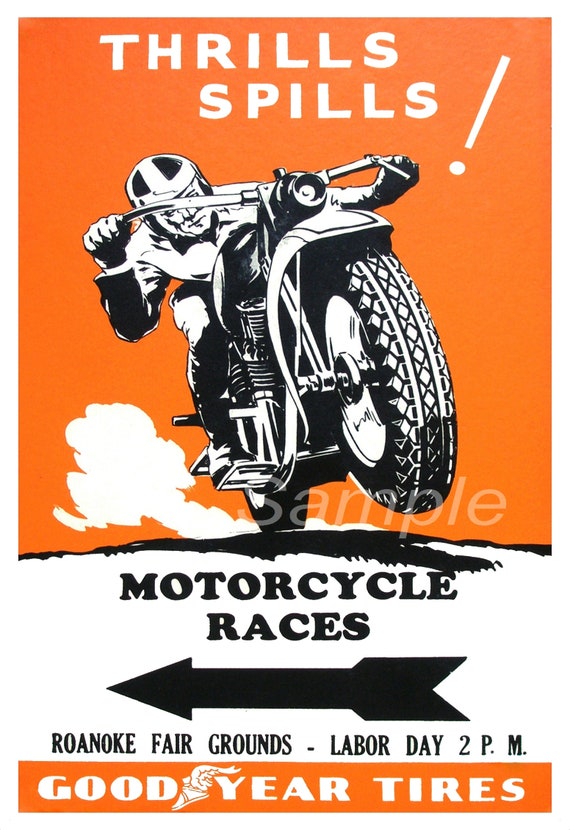This vintage-style flyer advertises motorcycle races at the Roanoke Fairgrounds on Labor Day at 2 p.m. The illustration predominantly features black, white, and a vivid orange color scheme. At the top, "Thrills! Spills!" is displayed in a bold, capitalized white font with an exclamation mark slightly askew. The main image depicts a black and white drawing of a motorcycle rider, helmeted and leaning forward, heading towards the right side of the image, creating an impression of motion towards the viewer. His face is partially obscured by the handlebars, and there are stylized clouds or smoke in the background. Beneath the rider, "Motorcycle Races" is written in a bold, black font on a white background, accompanied by an arrow pointing to the left. Below this information, the details "Roanoke Fairgrounds, Labor Day, 2 p.m." are presented in black lettering. The bottom section features an orange rectangle with "Goodyear Tires" boldly displayed in white font, alongside the Goodyear logo. The style is reminiscent of advertisements from the 1940s or 1950s, and there is a "sample" watermark superimposed on the image.